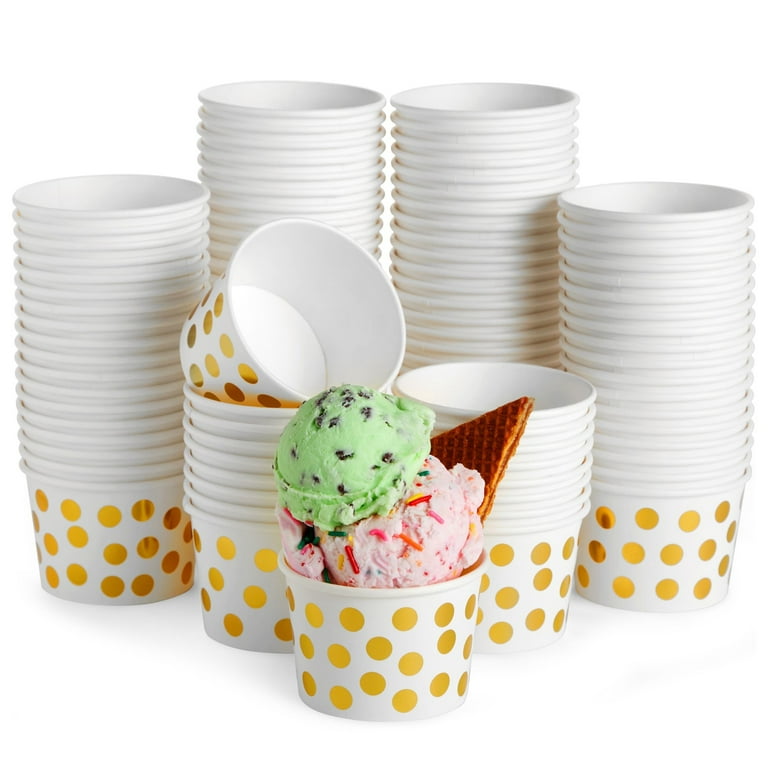The image displays a collection of small, white ice cream cups adorned with gold polka dots, stacked into six neat piles against a plain white background. One of the stacks features a cup that is tilted sideways. In the foreground, a single cup stands out, containing a scoop of strawberry ice cream topped with rainbow sprinkles and a scoop of green pistachio ice cream. A triangular waffle cone peeks out from under the strawberry scoop, adding a decorative touch. The remaining cups are empty and piled together, highlighting the singular filled cup amidst the orderly stacks.